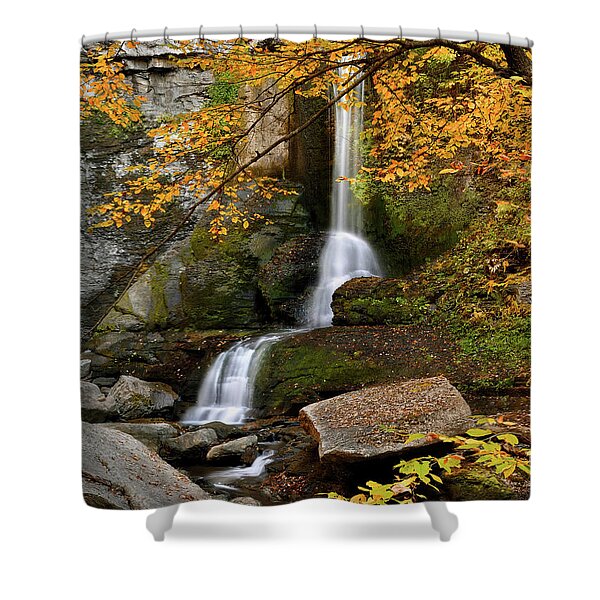The image displays a highly detailed shower curtain, resembling a realistic photograph, hanging from a long white shower rod with silver rings. The shower curtain features a captivating design of a waterfall in a fall-themed outdoor scene. The waterfall, captured through a long exposure technique, appears ethereal and misty, with white, ribbon-like water cascading over a rocky cliff and flowing into a small brook or stream surrounded by large rocks. The scene is enhanced by vivid fall-colored leaves in shades of yellow and orange, along with small patches of greenery. The bottom of the image reveals light gray legs of a bathtub, complete with drop shadows, adding a finishing touch to this serene bathroom setting.